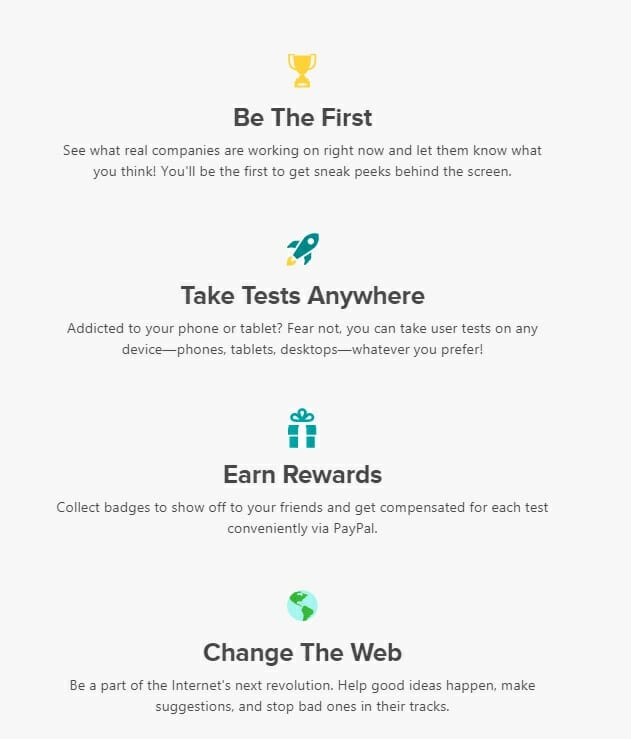This image is a screenshot of a website with a background in shades of gray. 

At the top, a prominent yellow trophy icon is accompanied by the bold text: "Be the First. See what real companies are working on right now and let them know what you think. You'll be the first to get sneak peeks behind the screen." 

Below this, a rocket icon introduces the text: "Take Tests Anywhere. If you're addicted to your phone or tablet, fear not. You can take user tests on any device – phones, tablets, desktops, whatever you prefer."

A gift box emblem follows, with the message: "Earn Rewards. Collect badges to show off to your friends and get compensated for each test conveniently via PayPal."

Finally, a globe icon highlights: "Change the Web. Be a part of the internet's next revolution. Help good ideas happen. Make suggestions and stop bad ones in their tracks."

The website appears to be a platform that enables users to participate in user testing for companies, earning rewards and compensation through their feedback.